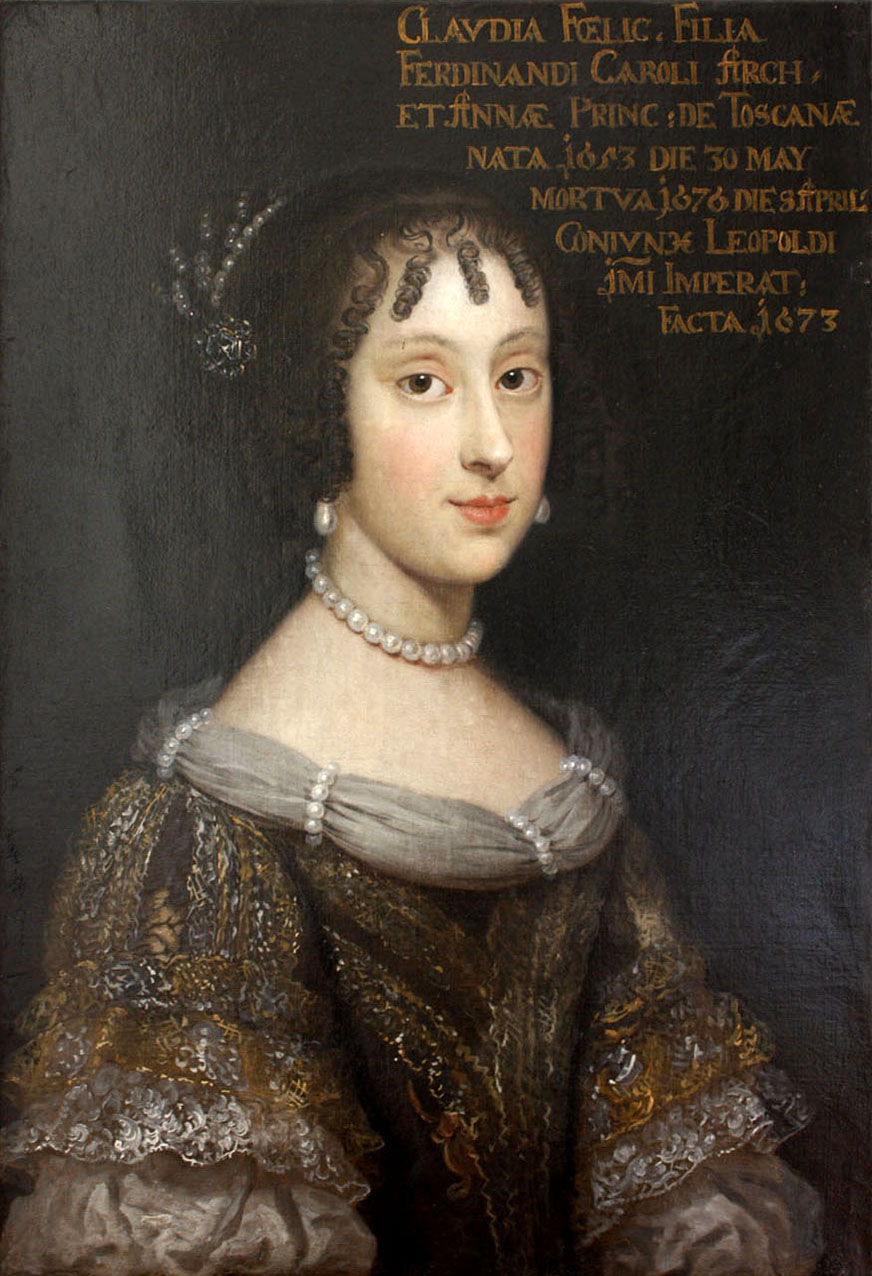This is a richly detailed color oil painting portrait, likely from the Renaissance period, titled "The Portrait of Claudia Felicitas" by Sebastiano Bombelli. The painting, set against a gray backdrop, features a stately young woman of around 30 years, occupying three-quarters of the image from head to elbows. She wears an elaborate brown and gold embroidered gown, adorned with a gray gathered ruche around the neckline interspaced with bands of white pearls. Her attire includes a white pearl choker, two teardrop-shaped white pearl earrings, and fluffy golden sleeves approaching the elbow. The subject has dark hair styled in a bun with an ornamented headpiece, and several dark brown ringlets cascade over her forehead. She has a fair complexion, brown eyes, and red lips. Text in an orange handwritten typography in the upper right corner of the painting identifies her as Claudia Felicitas along with references to other names, likely describing her lineage. The artwork reflects the meticulous craftsmanship and ornate fashion characteristic of the era.